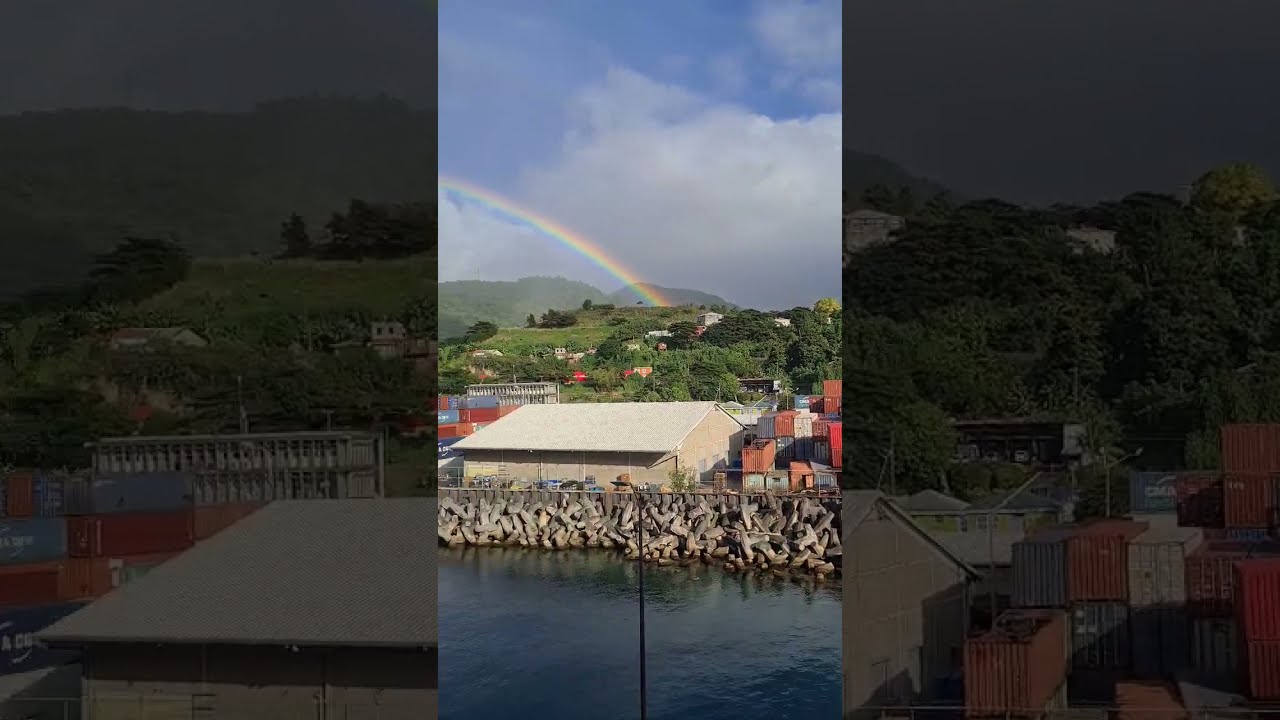The image is divided into three vertical segments, with the central portion being a vivid photograph and the side segments showing an enlarged, darker-colored detail from this central image. In the primary section, a serene body of blue water occupies the lower part, bordered by an extended pile of logs or brown tubes that form a barrier in front of a shoreline filled with buildings. Front and center is a large, one-story, beige-colored warehouse-like building, which looks to be made of wood and has stacks of assorted metal cargo containers to its right. The middle section of the image is rich with natural scenery featuring multiple layers of green hills adorned with trees. The backdrop includes softly dimmed hillsides that rise to meet a horizon where a vivid blue sky takes up around 40% of the frame, dotted with fluffy white clouds. Adding to the picturesque quality, a vibrant rainbow arcs from the left side, extending towards the middle over the hills. The detailed background also features bushes and shrubbery, enhancing the lush, verdant quality of the landscape.